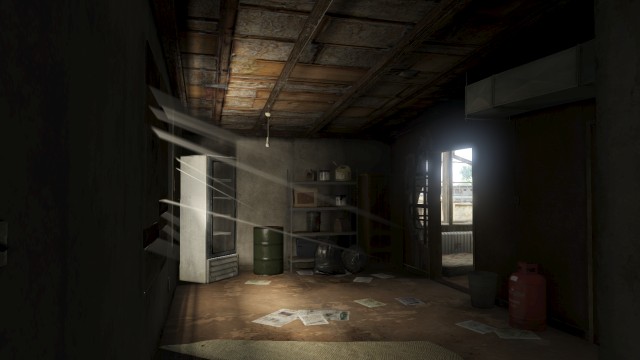The image is a screenshot from a video game depicting a grimy storage room. The ceiling is dilapidated, lacking drywall and exposing structural elements. On the right side, there is an open door letting in natural daylight, indicating a sunny day outside. The left side features windows with blinds, allowing additional light streams into the room. In the background, a gray, four-tiered shelf is visible, accompanied by a green barrel positioned to its left. Further left, a white refrigerator with a clear front panel stands, adding to the cluttered, utilitarian atmosphere of the room.